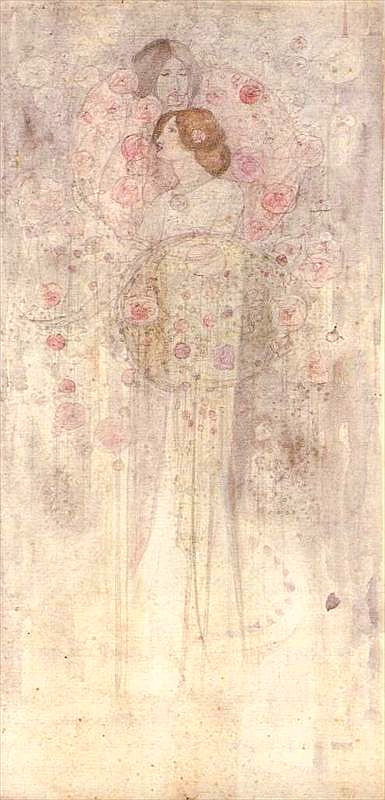The image depicts a very light-colored, almost faded scene with muted tones of light tan, pink, and brown. Central to the image is a sketch of two people, predominantly outlined with some filled colors, particularly in their hair. The woman in the foreground has bright brown hair swept into a bun and is wearing a floor-length white gown, giving the scene a bridal appearance. Surrounding her are faint, light purple and pink flowers, adding to the ethereal, wedding-like ambiance. The second figure, standing behind her, appears to be a woman with darker brown hair, looking down at the first woman's hair. This illustration has an overall faded, almost damaged quality, with hints of discoloration and mold-like gray areas, making the details appear less distinct. The bottom part of the sketch has a bright yellow glow, adding to the dreamy, vintage-like effect. Despite its worn-out look, the image evokes a sense of delicate beauty, reminiscent of an old, treasured wedding photograph with splashes of red and pink possibly representing flowers.